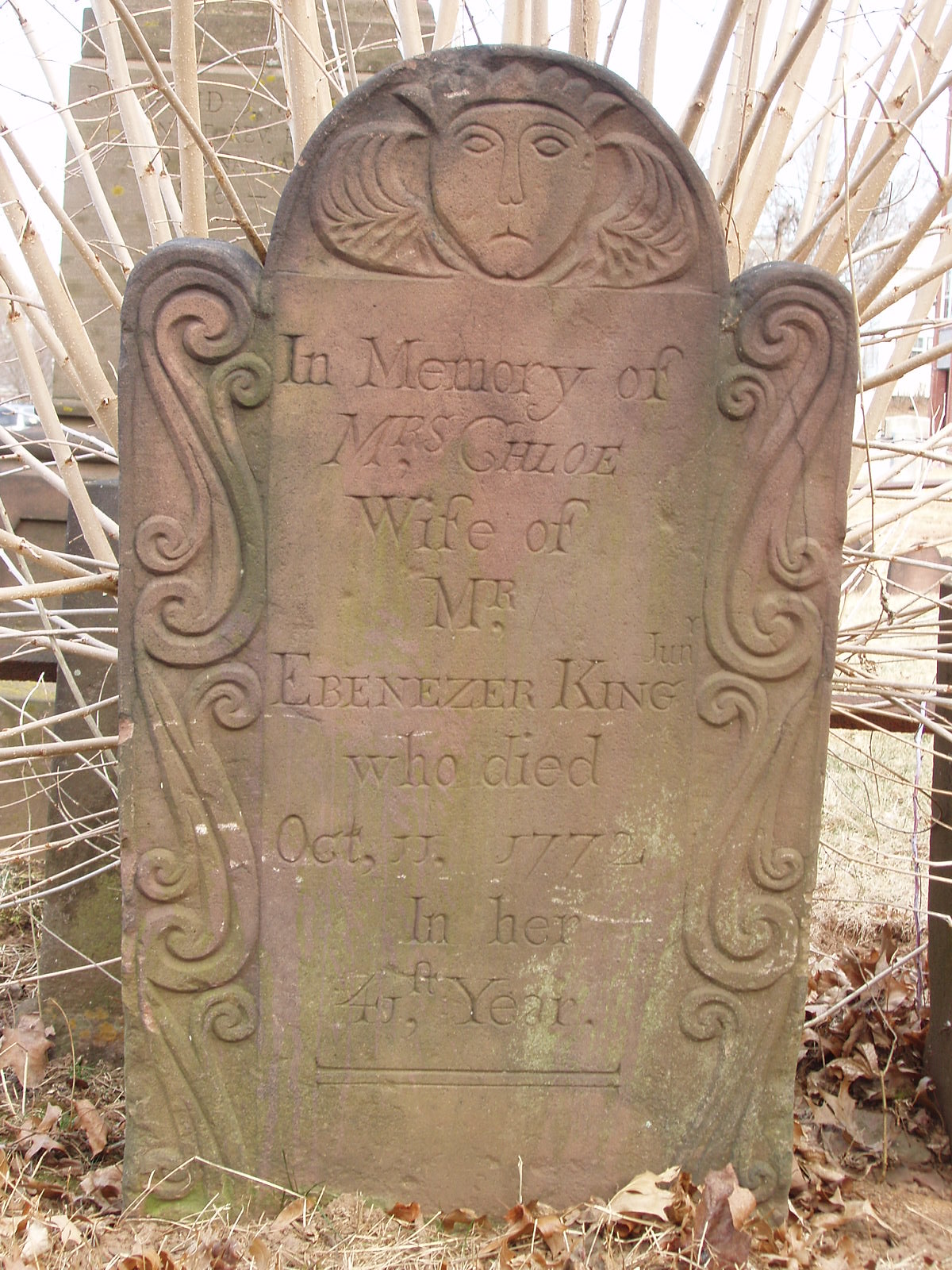The image captures an outdoor scene featuring an old colonial-era gravestone standing upright. It prominently displays an intricately carved face with wings and a crown at the top, alongside swirling designs etched into its sides. The gravestone bears the inscription: "In memory of Mrs. Chloe, wife of Mr. Ebenezer King, who died October 11th, 1772 in her 41st year." Surrounding the gravestone, there is a mixture of grass and dead leaves on the ground. In the backdrop, a tree with numerous white branches is visible, and another gravestone lies in the distance. The photo is taken in daylight, offering a clear and bright view of the scene with a portion of the sky visible at the top. The overall quality of the image is high, providing a detailed and sharp look at the historic gravestone and its surroundings.